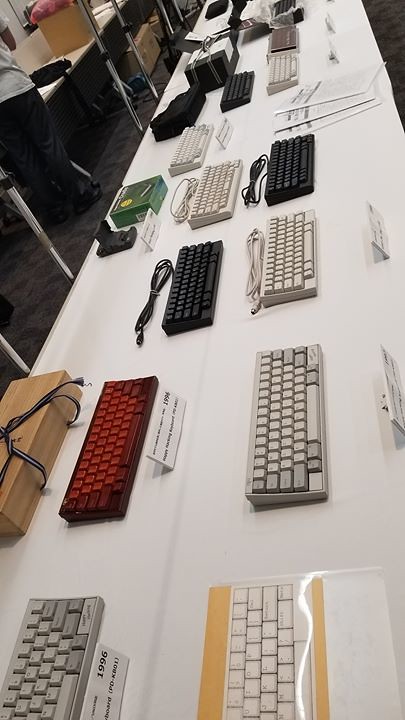The image captures a slightly overhead view of a long white table laden with an assortment of computer keyboards in various colors, including orange, gray, white, red, and black. Each keyboard has a descriptive white placard in front of it, with some indicating the name of the manufacturer and the year, such as 1996, though the rest of the text is not clearly legible. Several of the keyboards have their cords trailing behind them. Additionally, there are other items on the table, such as a green box and scattered pamphlets or papers, particularly towards the far end. In the top left corner of the image, a few black computer monitors can be seen, hinting that this may be an office or a store displaying computer equipment. The view includes a glimpse of someone's legs, and background elements appear to indicate a cubicle workstation setting. The photograph is shot in portrait mode, offering a comprehensive display of the items arranged neatly on the table.